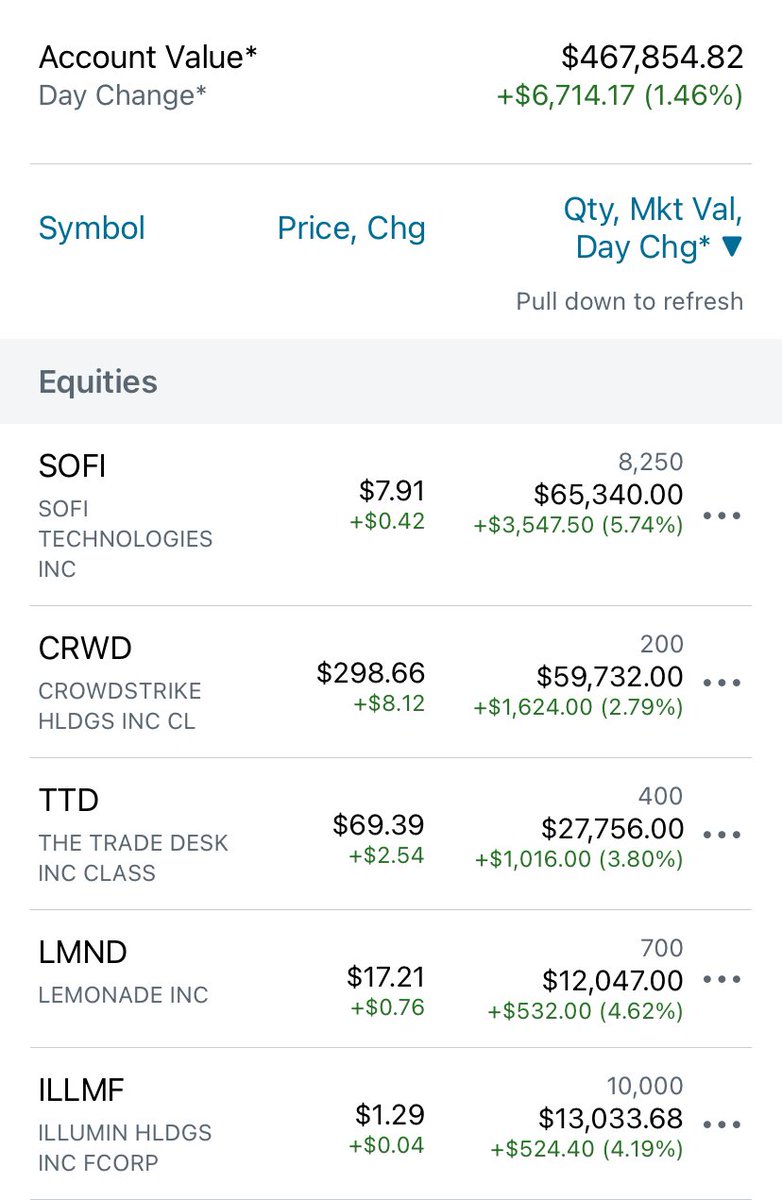The image depicts a detailed financial account summary showing a substantial total account value of $467,000. It highlights a daily gain of $6,700, representing a 1.46% increase. The account's investment portfolio includes several notable stocks such as SoFi, CrowdStrike, The Trade Desk, Lemonade, and Illumina Holdings. The largest holding is SoFi, with a current price per share of $7.91 and a total stock value of $65,000. The information is presented on a white background with black text, where positive changes are indicated in green, implying that negative changes would likely be shown in red. The text implies that not all investments are listed.